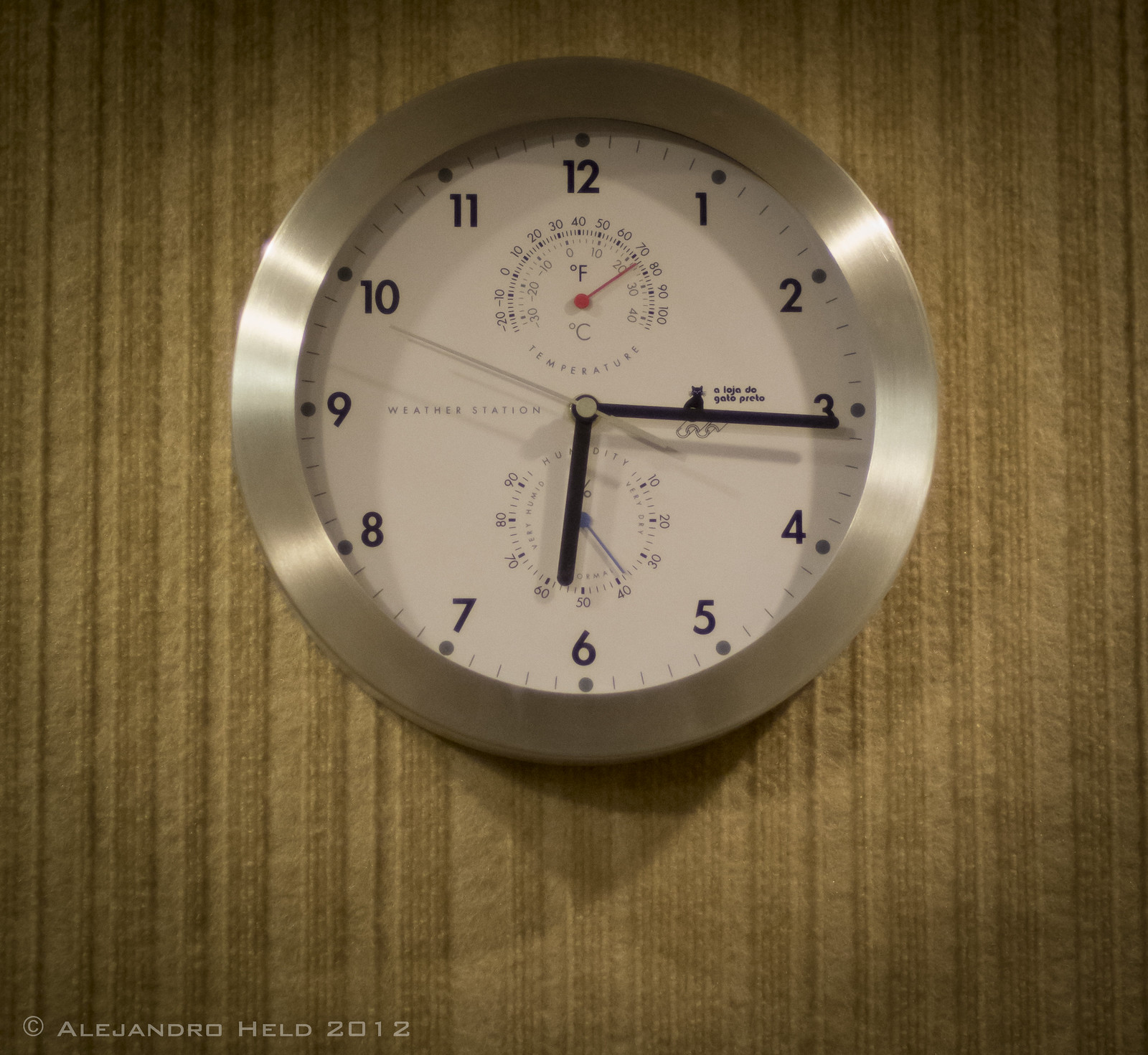The image features a detailed wall clock set against a distinctive background that resembles a carpeted or knit fabric with a yellowy-golden hue that almost crosses into green. Highlighted by its brushed silver rim, the clock showcases a traditional white face with hour and minute hands, indicating a time of approximately 6:16. The clock integrates a weather station functionality, with two smaller circles inside the main face: one below the 12 marking temperature in both Fahrenheit and Celsius, and another indicating humidity percentage. Between these circles, the text "weather station" is visible, flanked by the phrase "aloha de gato preto" on the right, accompanied by a tiny cartoon cat. Additionally, a small black cat accentuates the minute hand, and a copyright mark in the bottom left corner credits Alejandro Held, 2012.